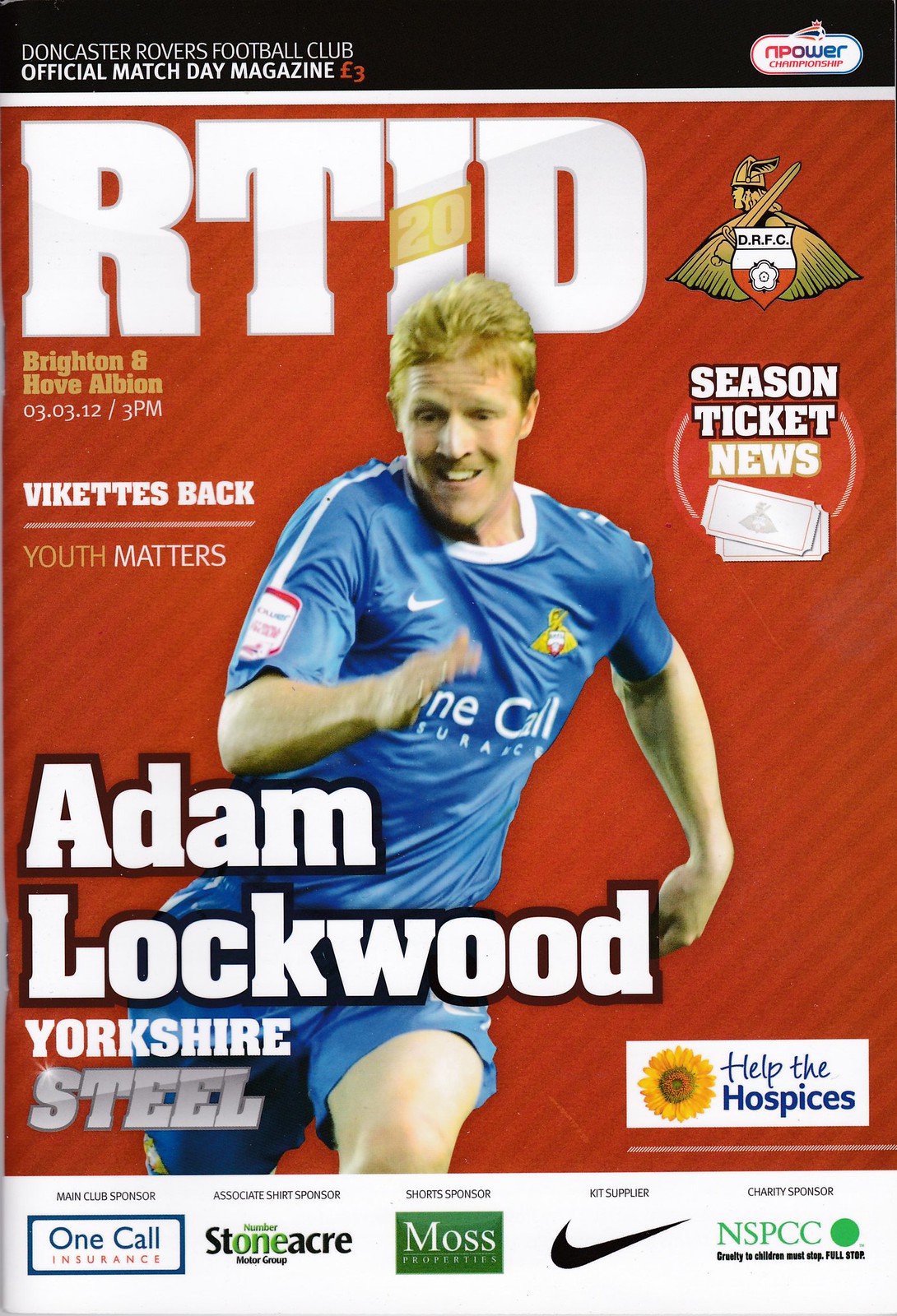This image is a detailed cover of a Doncaster Rovers Football Club Official Match Day Magazine. It features a thin black strip at the top with white text reading "Doncaster Rovers Football Club Official Match Day Magazine", alongside the price of "Three Pounds (£3)" on the right. Below this strip, there's a red background with diagonal gray stripes. Prominently displayed in large white letters is "RTID". Below this, in gold letters, it details the match information: "Brighton & Hove Albion 03-03-12, 3 p.m.", alongside the term "VIKETS".

In the center of the cover is an action shot of a player, Adam Lockwood, presumably in a soccer uniform, wearing a blue shirt and shorts. He's mid-run, with his right arm extended forward and his left arm slightly behind. Lockwood has short blonde hair and a mustache, and his intense focus is captured as he looks slightly downward. Across his midsection, in large white letters, is his name "Adam Lockwood", followed by "Yorkshire Steel".

To the right of him, the cover mentions "Season Ticket News". Also scattered across the cover are phrases like "Youth Matters" and "Help the Hospices", the latter accompanied by a small sunflower illustration. The bottom portion of the magazine has a white border featuring various advertisements, including recognizable logos such as Nike, One Call Insurance, Stoneacre Motor Group, Moss Properties, and NSPCC. An emblem appears in the right-hand corner, and the cover overall reflects the dynamic and vibrant essence of the match day.